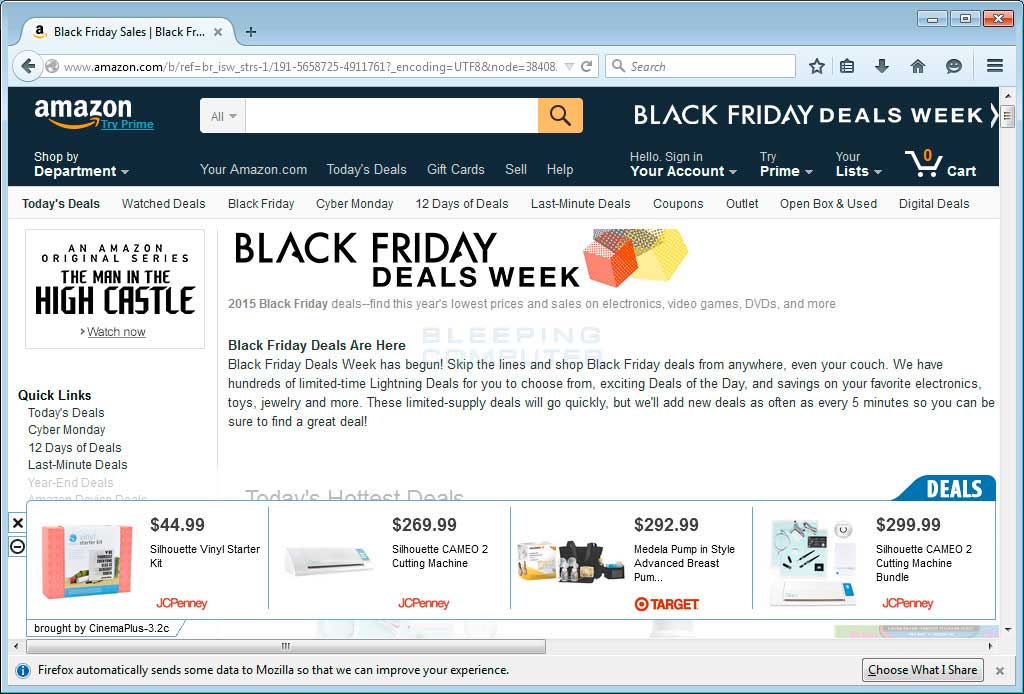**Detailed Caption for the Image:**

The screenshot showcases an Amazon website displaying their Black Friday sales. The top left of the page features the Amazon logo, recognized by the iconic gold arrow. The search bar prominently reads "Black Friday sales slash Black Friday" and the URL displayed is amazon.com. 

Users can search for products using the search bar or navigate through the site via a drop-down menu under "Shop by Department." The user is currently not signed in, as indicated by the "Sign in to your account" prompt. Additional navigation options include "Today's Deals," "Watch Deals," "Black Friday," "Cyber Monday," "12 Days of Deals," "Last-Minute Deals," "Coupons," "Outlet," "Open-Box," "News," and "Digital Deals." The shopping cart icon shows zero items.

In large, attention-grabbing letters, the page announces "Black Friday Deals Week," indicating that the sales event is in full swing. The main body of the site features colorful images of boxes in orange, yellow, and black hues, highlighting the 2015 Black Friday deals. The text encourages users to find this year's lowest prices on electronics, video games, DVDs, and more. 

The section emphasizes the ease of shopping by stating, "Black Friday deals are here. Black Friday Deals Week has begun. Skip the lines and shop Black Friday deals from anywhere [even from your couch]." It highlights that there are "hundreds of limited-time lightning deals" available, with new deals being added as often as every five minutes to ensure a variety of exciting options, particularly on electronics, toys, and jewelry. 

At the bottom of the page, a horizontal box showcases various deals from retailers like JCPenney and Target.